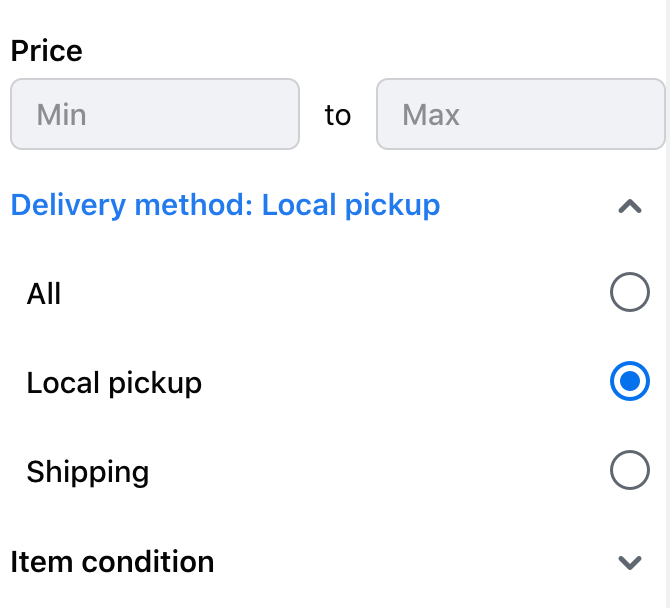This image captures a screenshot of a dialog box featuring multiple interactive components on a white background.

- **Top Left Section:**
  - The text "Price" is displayed in black.
  - Below this, there's a grey text box with the default text "min" in darker grey. Within this text box, the number "2" appears in black.
  - To the right of this is another grey text box with the default text "max" in darker grey.

- **Center Section:**
  - Below the price range, the words "Delivery method: Local pickup" are written in blue.
  - Adjacent to this text is a grey arrow pointing up and to the right, indicating a scrolling option.

- **Radio Buttons Section:**
  - Several radio buttons are listed under each other:
    - The first option is labeled "All" in black text on the left. Its corresponding round radio button on the right is empty.
    - The second option, "Local pickup," is listed underneath "All." This option’s radio button is selected, shown with a blue outer border, a white ring, and a blue center.
    - The third option, "Shipping," is displayed below "Local pickup" with an unselected and black-outlined radio button on the right.

- **Bottom Section:**
  - The words "Item condition" appear in black, with an arrow pointing downwards located at the bottom right corner, suggesting more options are available via scrolling.

This detailed description captures the layout and interactive elements present in the dialog box, indicating that additional options are likely hidden below due to the need for scrolling.